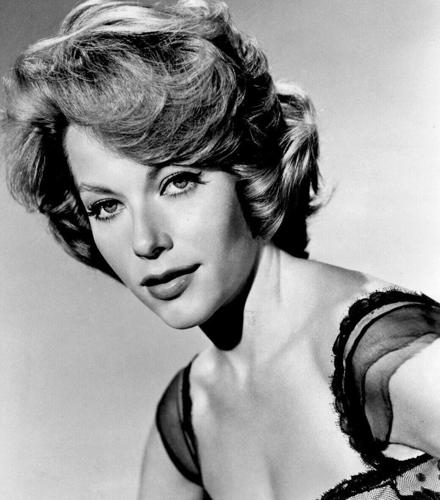This image is a vintage black-and-white publicity photo or headshot of a likely actress from the 1940s, 50s, or 60s, possibly Maureen O'Hara. The portrait captures a white woman with a light skin tone and distinct facial features. Her head is angled in the upper left corner while her shoulders and chest extend towards the bottom right corner of the frame. She has a short, wavy hairstyle that covers her ears and showcases retro curled bangs typical of the era. Her intense, suggestive gaze is directed straight at the camera, emphasizing her thick lips and expressive eyes. 

She wears a black lacy see-through garment, possibly lingerie or a nightgown, which features sheer black straps over her shoulders and delicate lace detailing around the chest area. Her neck and the visible parts of her arms are bare, giving the photo an elegant yet provocative aura. The background is a plain, very light gray or white, which makes her figure stand out prominently. The overall ambiance of the photo suggests it was taken indoors, focusing heavily on capturing the actress's facial expression and upper body details.